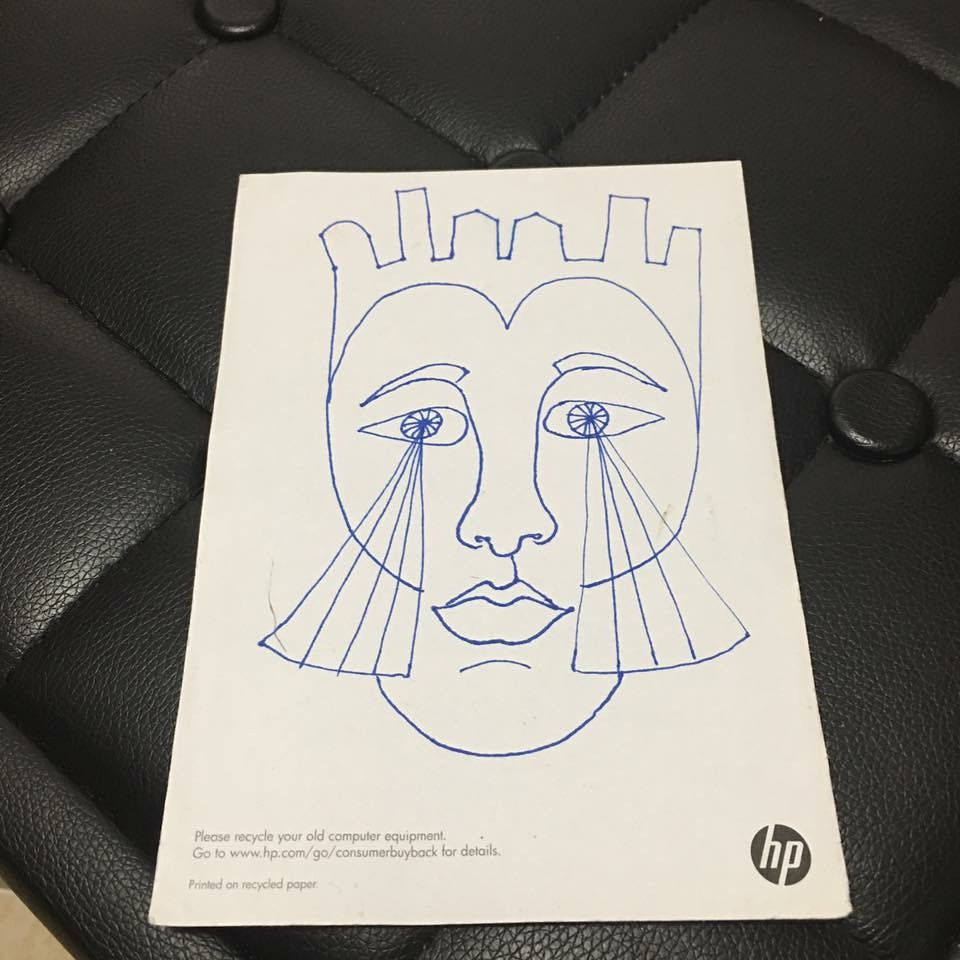This is a detailed description of a hand-drawn illustration on an 8.5" x 11" sheet of recycled Hewlett Packard paper. The drawing, executed entirely in blue pen, depicts a figure that resembles a king. Notably, the king’s crown is an outline of a cityscape, featuring curved skyscrapers that arch above his face and down to a point, with two extensions curving over his eyes. The king’s facial features include defined eyebrows, eyes that are unshaded but emit four prism-like rays, a dimensional nose that meets the eyebrows, a pronounced cleft above the mouth, a thin upper lip, a fuller bottom lip, and a small chin. The sketch exhibits a degree of artistic skill, especially in the rendering of facial dimensions.

The paper is positioned on a black stool or chair upholstered in a leathery fabric, textured in a square pattern with round buttons securing it. Behind the drawing, the printed message reads, "Please Recycle Your Old Computer Equipment. Go to www.hp.com/go/consumers andenbuy back for details," along with "Printed on Recycled Paper" and the Hewlett Packard logo located on the left-hand side.

The meticulous pen work, combined with the recycled medium, suggests it might be the back of a Hewlett Packard manual.